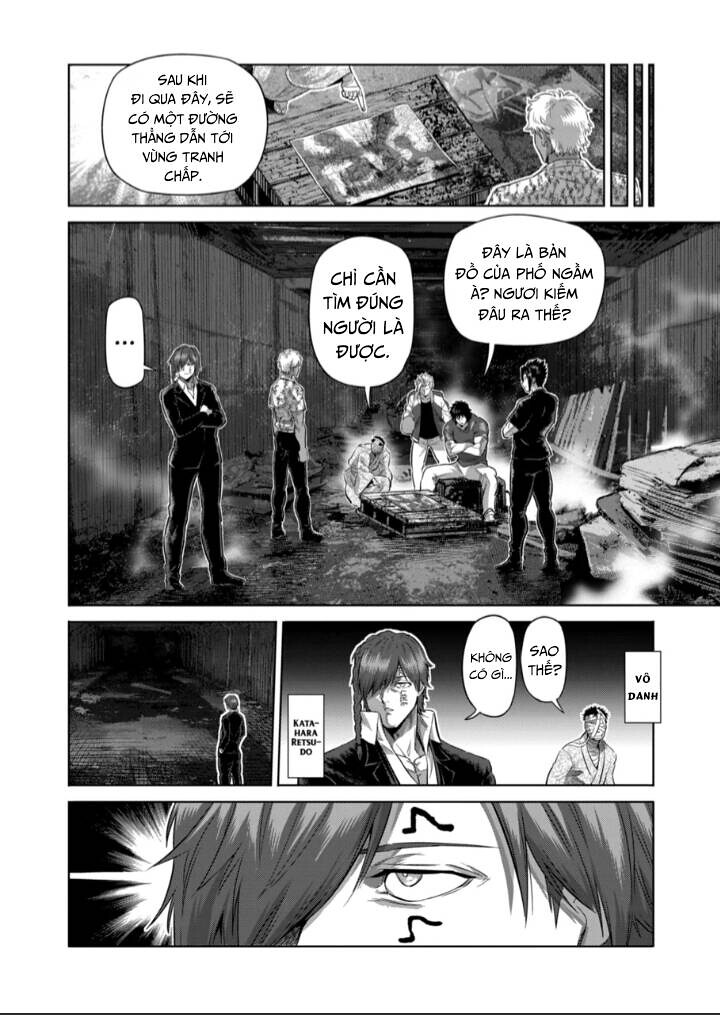A gray-toned manga page featuring four vertically arranged panels. The topmost, narrow panel depicts the back of a man with short hair, leaning over a table with a map on it. Another hand is shown pointing at a specific spot on the map, accompanied by a dialogue bubble in an unidentified Asian language.

In the larger, second panel, several people stand in what appears to be a dimly lit room or a warehouse. To the left, a person with crossed arms has a bubble with an ellipsis. To their right, a person sits next to an indistinct central object, engrossed in conversation with others standing around. Dialogue bubbles are scattered throughout, indicating an intense discussion or planning session.

The third, thinner panel shows an exterior scene with clouds, a person on the left standing, and another figure with ponytails and a suit depicted more closely on the right. This figure has a speech bubble and a narrative box surrounding them, contributing to the ongoing dialogue. A more distant individual gazes towards the viewer.

The final, bottom panel zooms in on the face of a character, drawing attention to their intense eye. Hair partially covers the face, with noticeable tattoos or marks above and below the eye. The dark background behind them suggests they are noticing something significant.